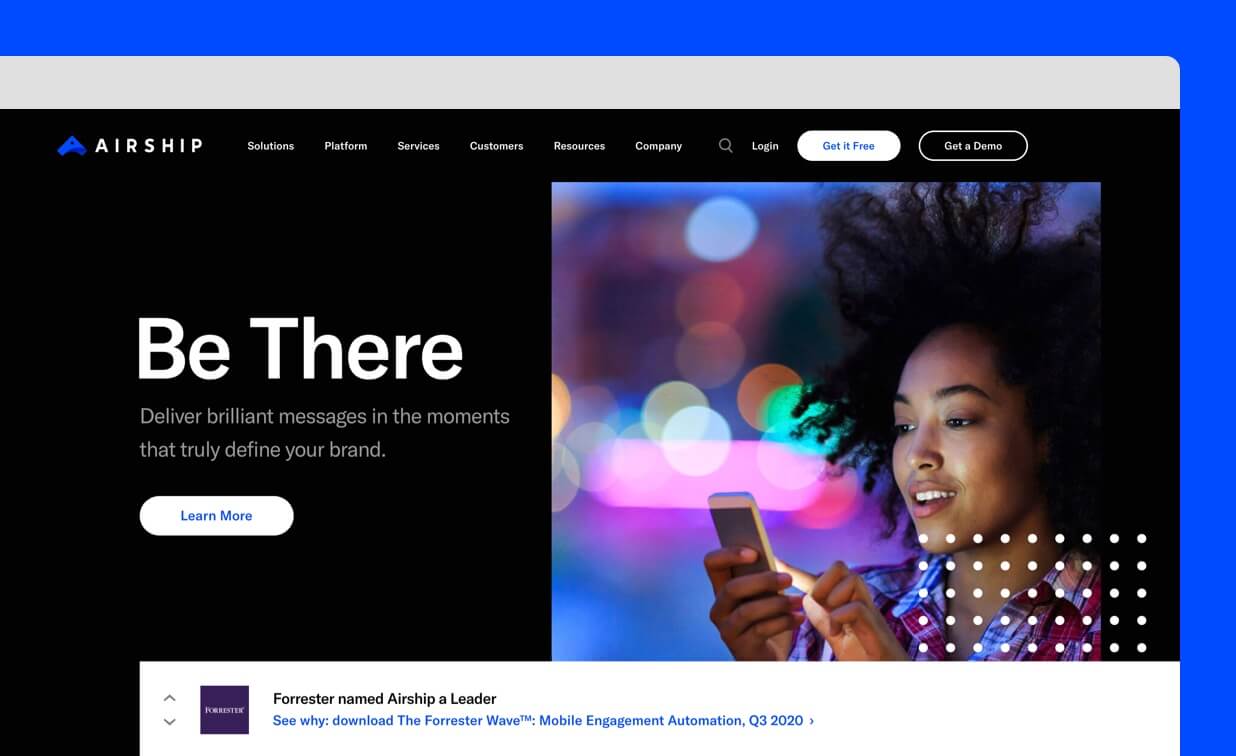Below the primary black website header, there's a blue background strip intersected by a gray bar at the top. The remaining background is predominantly black. To the right, there are six buttons arranged horizontally, accompanied by text that describes their functionality. One of the buttons highlights an easy access to obtain a demo. Notably, the final buttons in the row are distinctly white and black, respectively. Beneath these, a prominent Excel menu is displayed, primarily showing the 'View' tab, which contains several text options for deliverables. The interface appears unique to the brand depicted. The entire layout is captured in a square-shaped image, with an overlay note on a phone, detailing a special offer.